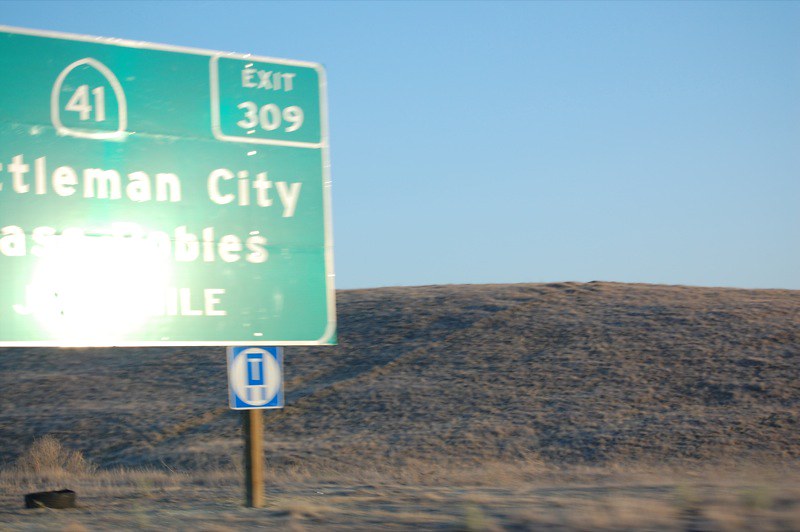This photograph, taken from the roadside, captures a large green highway sign partially obscured by a glare from the sun, indicating "Exit 309" in the top right corner. The sign, positioned at the side of the road, appears to be for a location named "T-L-E-M-A-N city," with a circled number 41 at the top. The bright reflection obscures the lower part of the sign where additional text is unreadable. Below the green sign, there is a blue and white sign featuring a blue box with a white T in its center. A single brown pole supports the sign on the lower right side. The backdrop reveals an arid, sloping hill, sparsely covered with brown grass and hints of green vegetation, extending up to the horizon against a clear, daylight blue sky devoid of clouds.